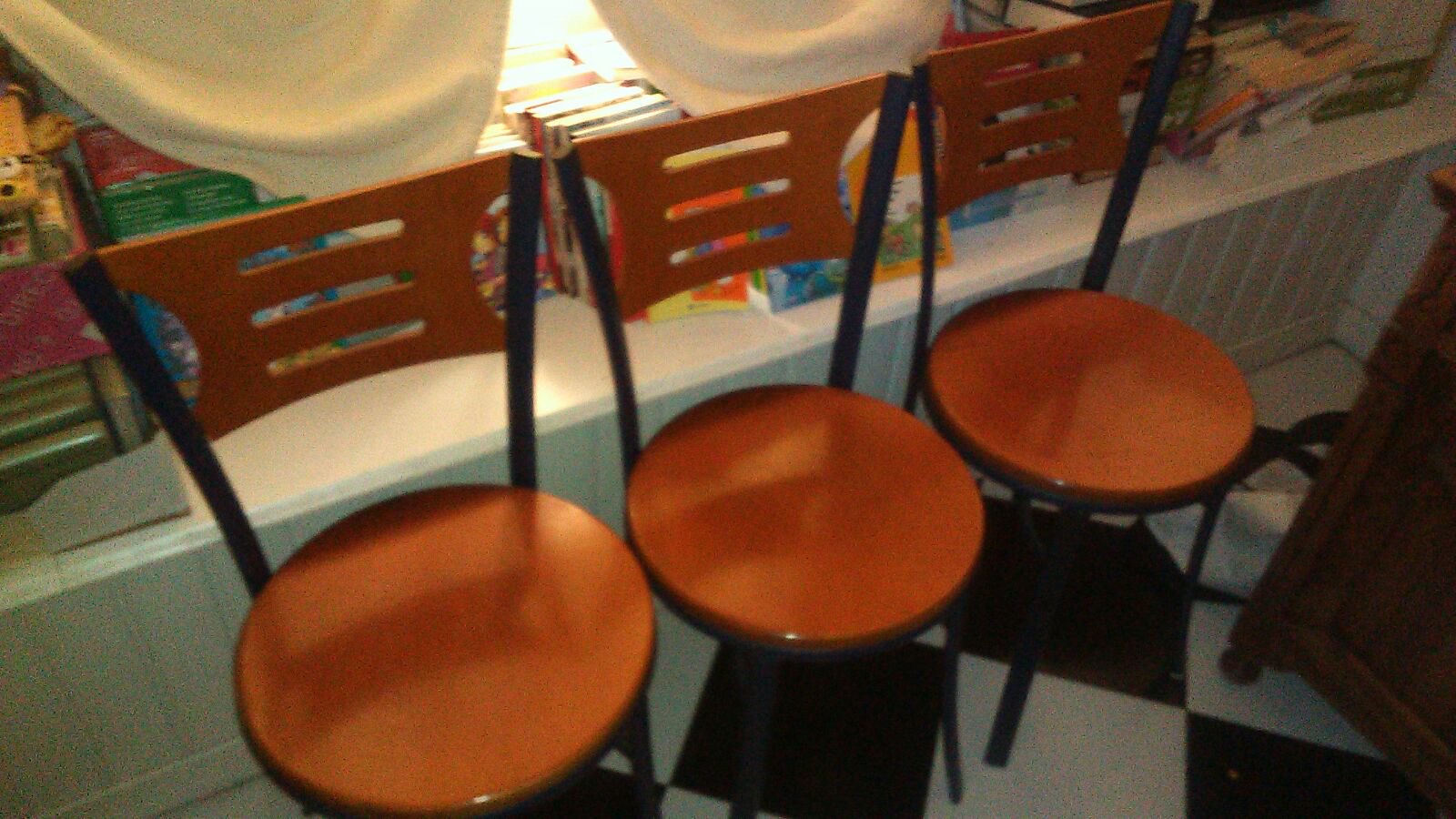The image depicts a trio of identical barstool chairs positioned on a black and white checkered floor. Each chair features a circular, tan-brown wooden seat and a matching wooden backrest supported by two black metal poles that extend down to form the back legs, while the front legs are also black. They are likely designed for use in a waiting area, possibly in a restaurant or near a kitchen island or bar. Behind the chairs is a cluttered white shelf filled with various colorful objects, including books in shades of red, green, blue, white, orange, and yellow, though the titles are not discernible. At the top right corner of the shelf, there appears to be a partially visible brown drawer or dresser. Additionally, folded white curtains rest on top of the objects on the shelf, adding to the array of items behind the seating area.